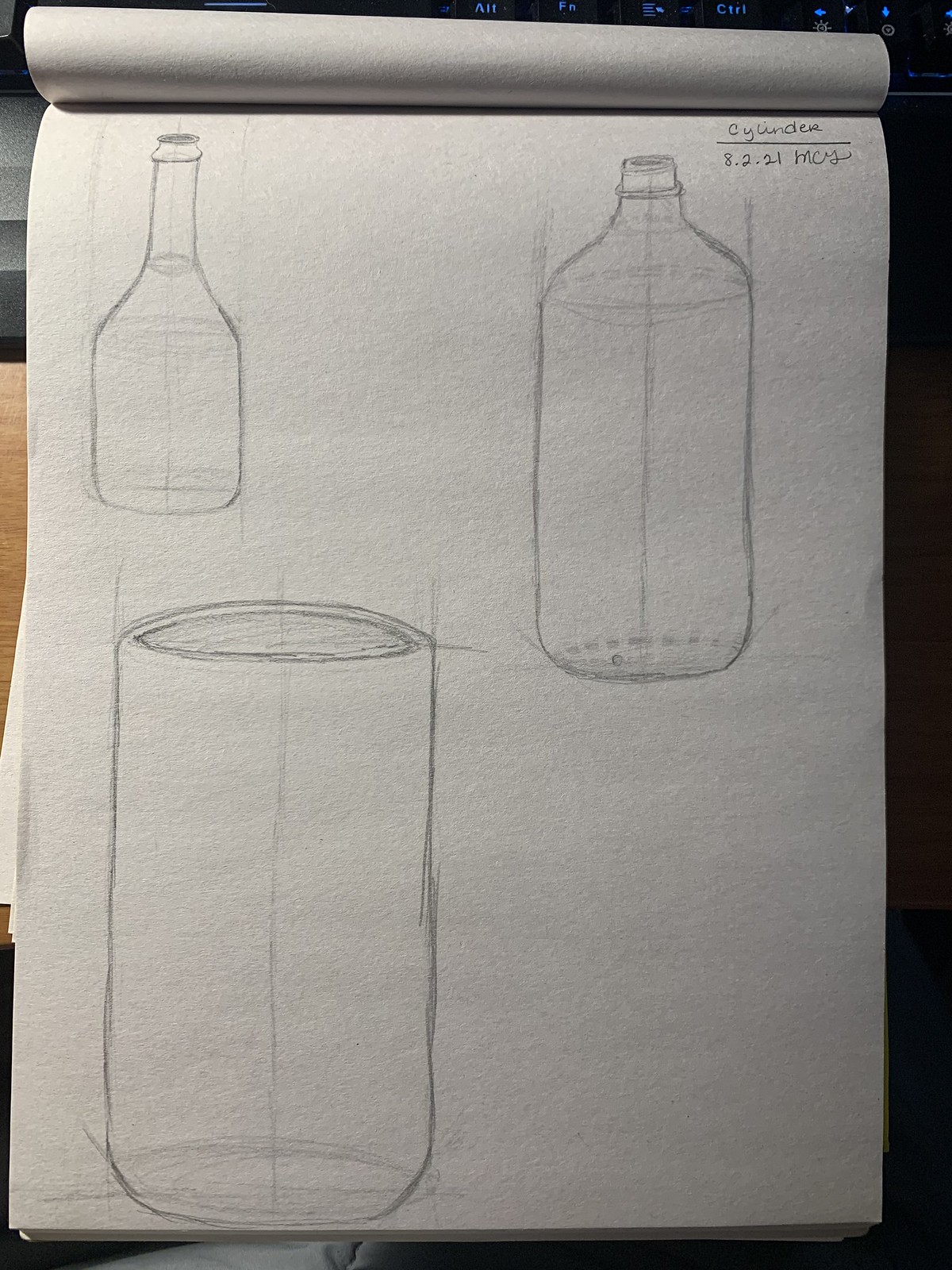The image captures a detailed pencil sketch on a white piece of paper within a sketchbook, partially covering a brown desk and keys from a keyboard illuminated with blue light. The sketchbook page, bound at the top, features a drawing practice focused on cylinders. Titled "Cylinder 8-21" and signed "MOS" by the artist, the drawings include three bottles and a glass. In the top left, an open bottle with liquid near the neck could resemble a salad dressing or vinegar bottle, showing marks where a label might go. The top right presents a taller, thicker bottle reminiscent of a ketchup bottle with a faint hint of threading at the neck. Below this bottle, a tall glass stands out. Additional drafting lines and erasures hint at the artist's process in refining proportions and shapes. In the bottom left, another cylindrical bottle appears unfinished, focusing on the broader base and midsection.